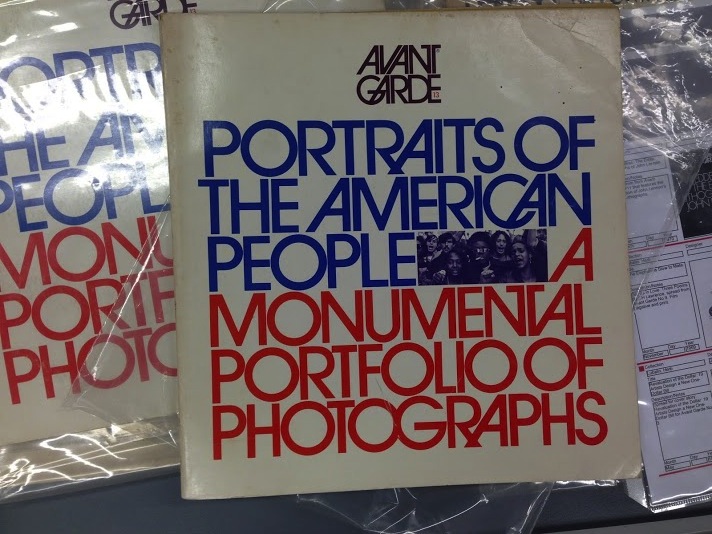In the landscape-oriented color photograph, the central focus is a square sticker with a white background, prominently placed in the middle of the frame. At the very top of the sticker, the logo "Avant Garde" is printed in black. Beneath this logo, centered in blue text, are the words "Portraits of the American People," followed by a narrow black-and-white photograph featuring the faces of diverse individuals, including some African Americans and Hispanic people. This imagery is bold and evocative, capturing the essence of a crowd with many individuals appearing to have their mouths open. Below the photograph, in red text, is the phrase "A Monumental Portfolio of Photographs," making the full title read: "Portraits of the American People, A Monumental Portfolio of Photographs." The text and image on the sticker are aligned to form a balanced, square shape. To the left of the main sticker is another identical sticker, still in its shrink-wrap packaging. On the right, partly covered by plastic, is a partially visible black-and-white document, adding to the sense of a display showcasing these items.